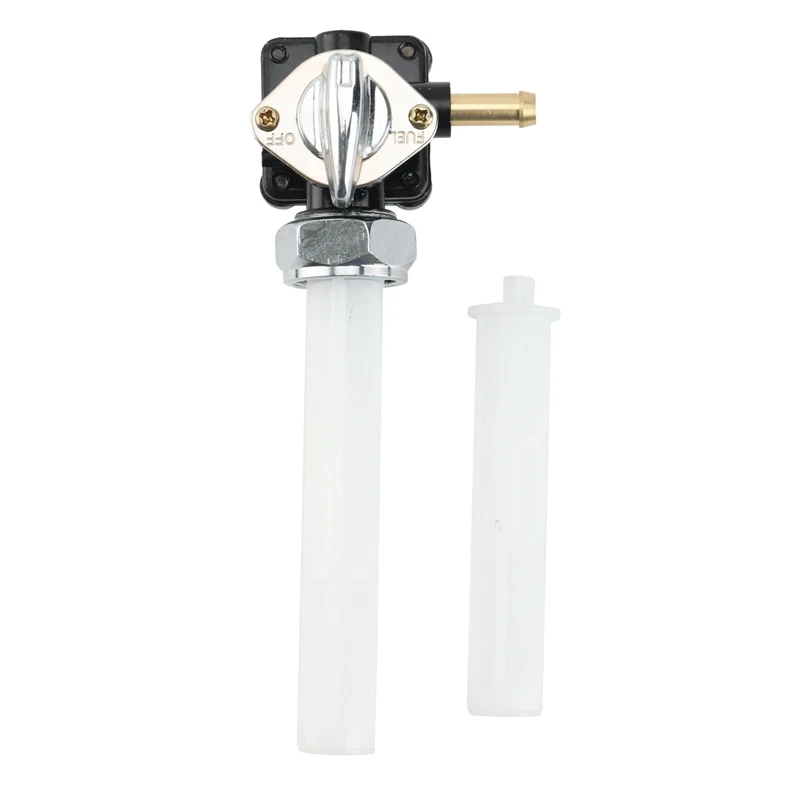The image features two white cylindrical tubes against a plain white background. On the left, a longer tube is topped with a silver bolt that's connected to a black plastic square. This square has a circular opening on the top right side and a lemon-shaped silver metal dial, with the words "FUEL" on the right and "OFF" on the left when viewed upside down, indicating the image is rotated. The dial is fastened with a screw on either side. Extending from the right of the square is a gold-colored metal pipe. Beneath the square, the white tube connects to the upper section via a large, adjustable screw. To the right in the background, a smaller white tube with a slightly projecting cap attaches a narrower tube at the top, measuring about a quarter of an inch in both width and height. The overall length of the longer tube is between three to four inches. The composition highlights the intricate metallic and plastic components of a nozzle and its attached parts.